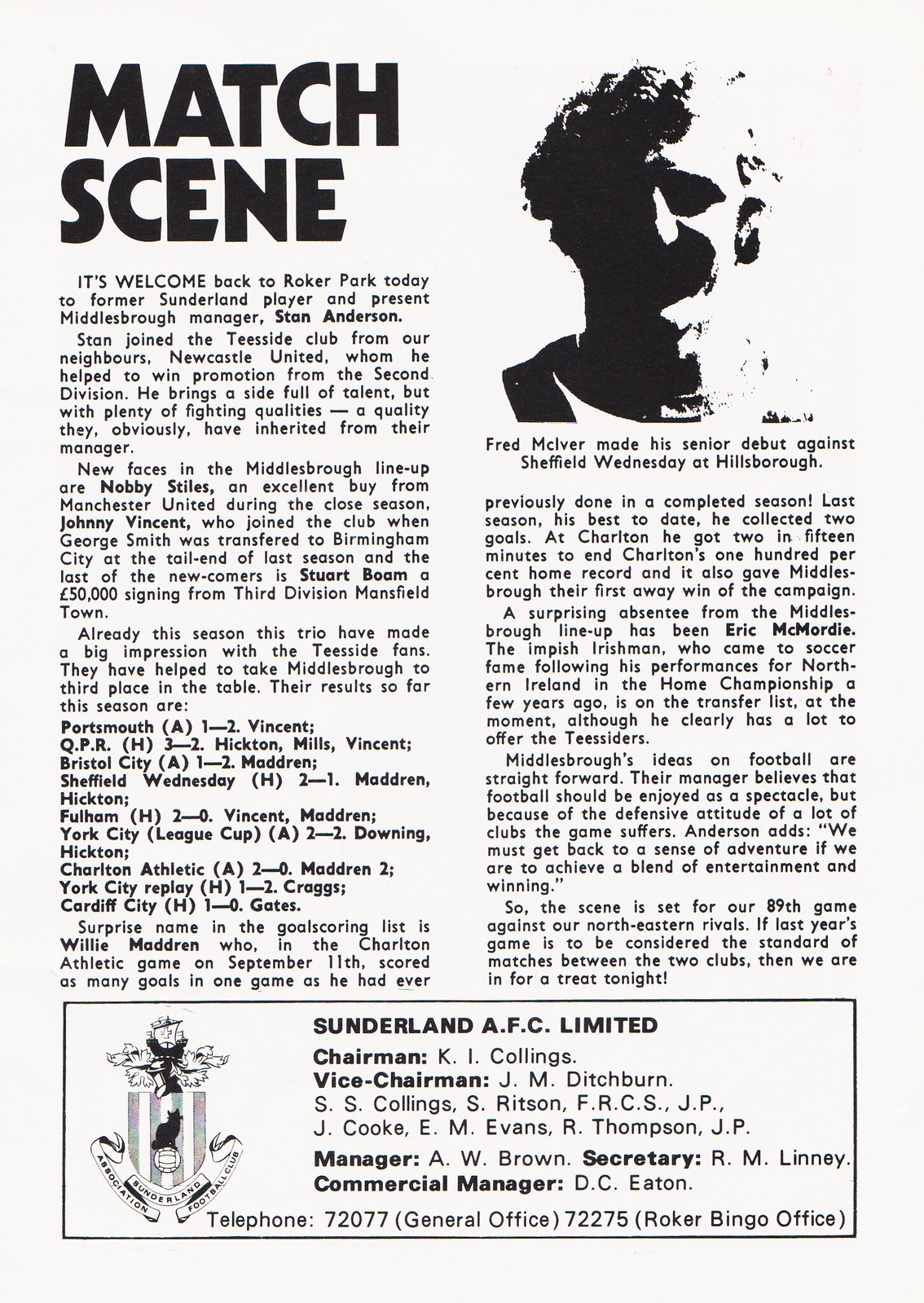This black-and-white image is a scan of a vintage program page from a soccer match, prominently featuring an article similar in style to a newspaper. The header at the top left reads “Match Scene” in bold black letters. The article welcomes back Stan Anderson, a former Sunderland player and current Middlesbrough manager, to Roker Park. The narrative highlights Anderson’s career journey, detailing his move to Middlesbrough from Newcastle United, where he contributed to winning a promotion from the second division.

The article is accompanied by a black-and-white headshot of Stan Anderson, though the quality is poor, obscuring clear details except for the basic hint of a jersey. The image is divided starkly, with one half in black and the other in white, making it challenging to discern more specific features of Anderson’s face or attire.

Below the article, encased in a separated box, is information about Sunderland AFC Limited, listing roles such as Chairman, Vice Chairman, Manager, Secretary, and Commercial Manager, along with two telephone numbers— one for the general office and one for the Roker Bingo office. The crest of Sunderland AFC is also included at the bottom of this boxed section.